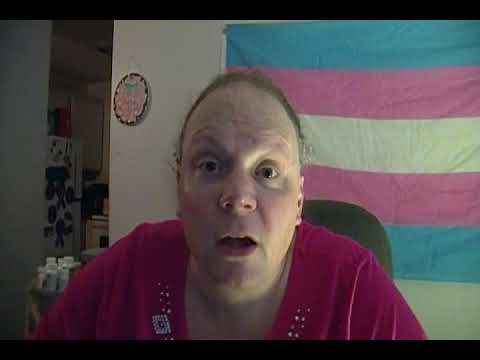The image depicts an older, light-skinned woman with rosy cheeks, possibly in her late 50s. She is slightly heavyset and is wearing a hot pink shirt adorned with silvery rhinestones around the collar. Her blonde hair is tied back. The woman appears to be speaking into a computer camera, mouth slightly open, showing her top two teeth, giving her an expression of surprise or mid-speech.

Behind her, a turquoise, pink, and white striped flag—identifiable as the transgender pride flag—hangs on the wall. Adjacent to the flag, there is a circular piece of artwork with light pink hues. The room around her is dimly lit, and she is seated in a black computer chair. In the background to her left, an opening leads to what seems to be a kitchen area.